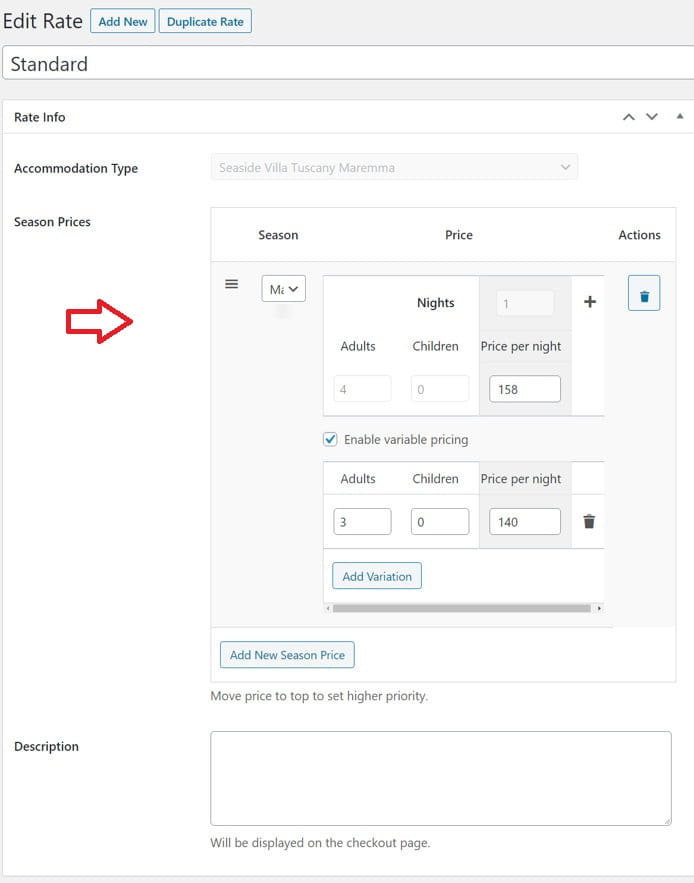The image depicts a comprehensive webpage interface mostly set against a white background, with a gray header at the top. In the top left corner, the text "Edit Rate" is displayed in black. Adjacent to this, there are two blue-rimmed buttons with gray backgrounds and blue text: the left button reads "Add New" and the right one says "Duplicate Rate." Below these buttons is a long white bar with the word "Standard" aligned to the right in black text.

Underneath, there is a white section labeled "Rate Info" on the left. On the far right, this section features two gray 'V' icons (one pointing up, one pointing down) and a triangle pointing up, suggesting an expandable section below.

In the ensuing large white area, "Accommodation Type" is written in black on the right. Directly below this text is a grayed-out dropdown box containing the options "Seaside Villa, Tuscany, Mirama," that is currently not clickable. Beneath this, there is a heading labeled "Season and Prices" in black, with a red arrow pointing right towards a detailed, multifaceted options box.

At the top of this options box, a white bar hosts the headers "Season," "Price," and "Actions" in black text, followed by a gray section featuring three horizontal black bars in the upper left corner and a dropdown menu labeled "MR."

Directly below is a section divided into two parts: the left side is labeled "Adults" with a grayed-out box showing the number '4,' and the right side is labeled "Children" with another grayed-out box showing '0.' Another grayed-out section indicates some variable element, displaying the number '1.'

Further down is the label "Price Per Night" in black, succeeded by a box showing '158' in black text. To the right is a thin white bar with a black plus sign. Below, a checkbox marked with a blue check reads "Enable Variable Pricing," and a thinner box shows the same variables as prior sections. The "Adults" section now displays '3,' the "Children" section is highlighted in blue and shows 'blue,' while the "Price Per Night" box now shows '140.' To the right of the price, there is a trash can icon.

Beneath this, a pale blue button with "Add Variation" inscribed in blue text is displayed, accompanied by a scroll bar at the bottom with limited scrollable area.

In the lower-left portion, a white area contains another long box with blue letters that read "Add New Season Price." Separately, a blue-rimmed box with a blue trash can icon is located to the top right. Below the extensive options box is an instruction in black text: "Move Price to Top to Set Higher Priority." In the lower left, the text "Description" in black precedes a large, empty text box. Below this, a message in black reads, "Will Be Displayed on the Checkout Page."